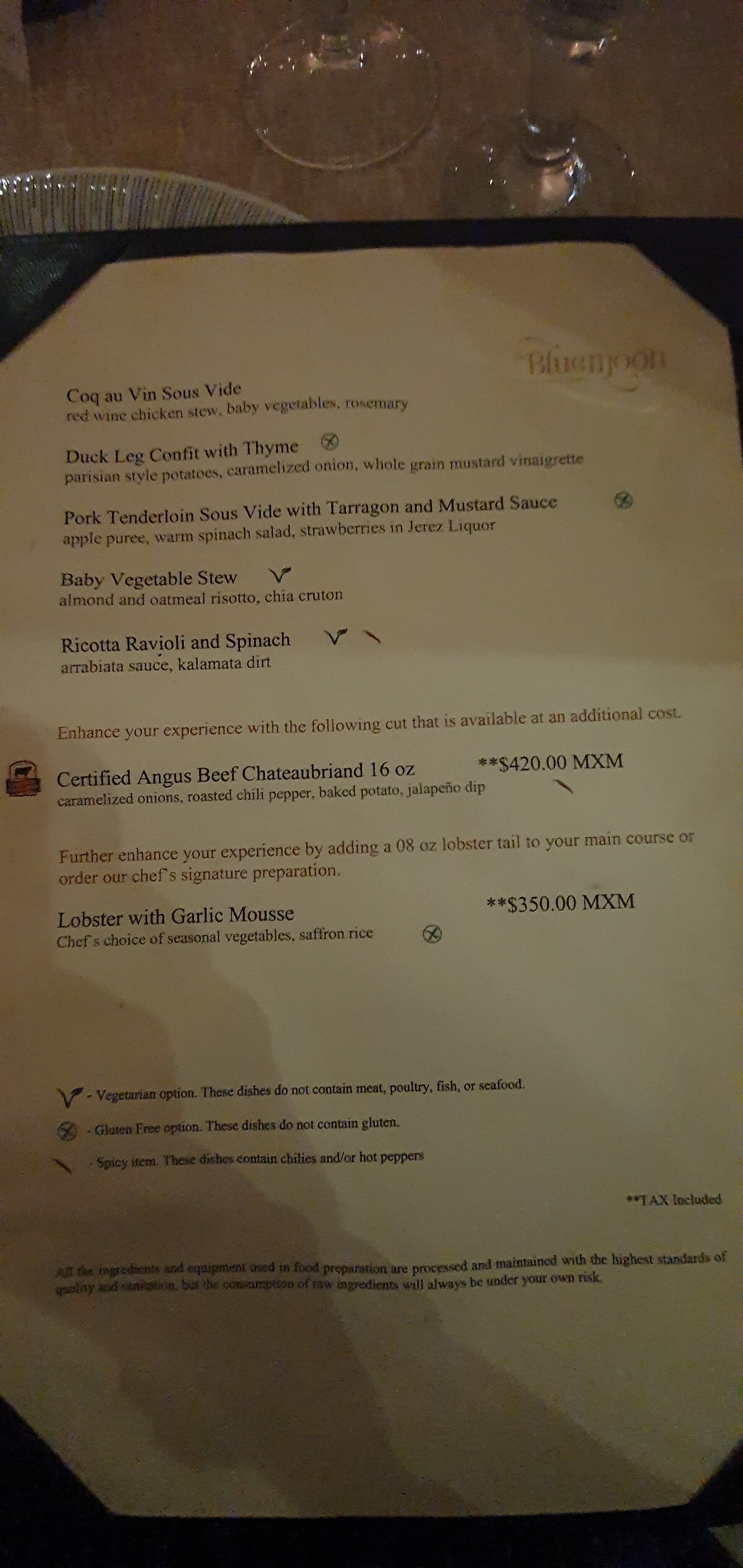This is a detailed photograph of a sophisticated menu from a dining establishment. The menu itself is crafted on a white backdrop, bordered with black edges and outlined in black, giving it a sleek and polished look. At the top right corner, the menu proudly displays a logo that reads "Blue Moon."

The menu features a selection of gourmet dishes including:

- Coq Au Vin Sous Vide
- Duck Leg Confit with Thyme
- Pork Tenderloin Sous Vide with Tarragon and Mustard Sauce
- Baby Vegetable Sous
- Ricotta Ravioli and Spinach

Below these items, an invitation encourages diners to "Enhance your experience with the following cut available at an additional cost." The option listed is a:

- Certified Angus Beef Chateaubriand, 16 oz. priced at $420.00 MXM

Further enhancing the experience, the menu suggests adding an 8 oz. Lobster Tail to the main course or ordering the Chef's Signature Preparation, which includes:

- Lobster with Garlic Mousse for $350.00 MXM

To assist guests with dietary preferences and restrictions, the menu includes helpful icons and descriptions at the bottom. A leaf symbol denotes "Vegetarian Option," indicating dishes that do not contain meat, poultry, fish, or seafood. A circle with an X through it signifies "Gluten Free Option," ensuring these dishes do not contain gluten. Additionally, a slanted line marks "Spicy Item," indicating these dishes contain chilies and/or hot peppers.

At the very bottom, there is a smaller, nearly unreadable text mentioning all the ingredients and equipment used in the preparation. The menu is subject to considerable shadows, particularly concentrated at the bottom left corner. The top of the image reveals a table setting in the background, complete with two glasses, adding context to the dining ambiance.